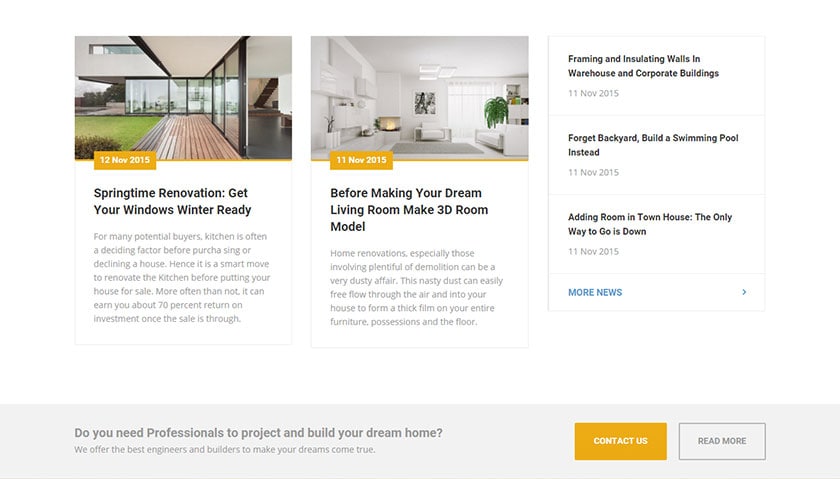This is a detailed screenshot from a property improvement and homebuilding website. The webpage features a simple, clean design with a white background and is highlighted by two prominent images. The first image showcases the exterior of a modern residential building, while the second captures the interior of a stylish living room. Both images serve as links to articles, with the exterior image dated November 12, 2015, and titled "Springtime Renovation: Get Your Windows Winter Ready." This article advises on preparing windows for the winter season. The living room image is dated November 11, 2015, and is titled "Before Making Your Dream Living Room, Make a 3D Room Model." It promotes the idea of creating a 3D model of a room prior to decorating or designing it in reality.

In addition to these two articles, the site offers text links to various other dated articles related to property renovation and decoration. These include topics such as "Forget a Backyard, Build a Swimming Pool Instead" and "Adding a Room in a Townhouse: The Only Way to Go is Down."

At the bottom of the website, there is an advertisement within a grey text box. The ad reads, "Do you need professionals to project and build your dream home? We offer the best engineers and builders to make your dreams come true." This section includes contact information and buttons labeled "Contact Us" and "Read More."

Overall, this website appears to serve as a comprehensive resource for home improvement, renovation, and building, with potential links to professional services offered by engineers and builders.